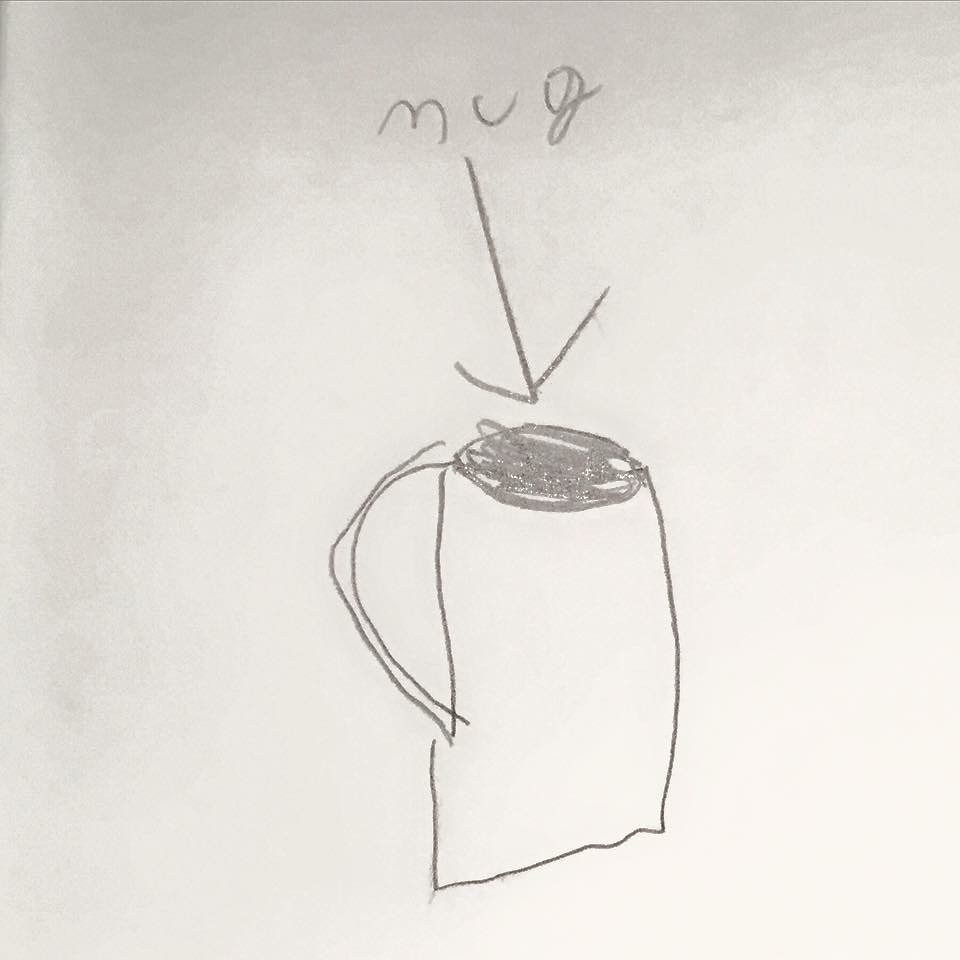A charming pencil drawing by a young child, estimated to be around seven or eight years old, depicts a simple yet endearing mug. The word "mug" is scribbled in adorable, childlike handwriting, with an arrow pointing towards the mug they have drawn. The mug itself is represented as a basic rectangle with an oval on top, skillfully shaded to appear full of liquid. Two semi-circles on the side cleverly illustrate the handle. This delightful artwork, complete with a beautifully formed cursive "G," is drawn on plain paper, showcasing the innocence and creativity of its young artist.